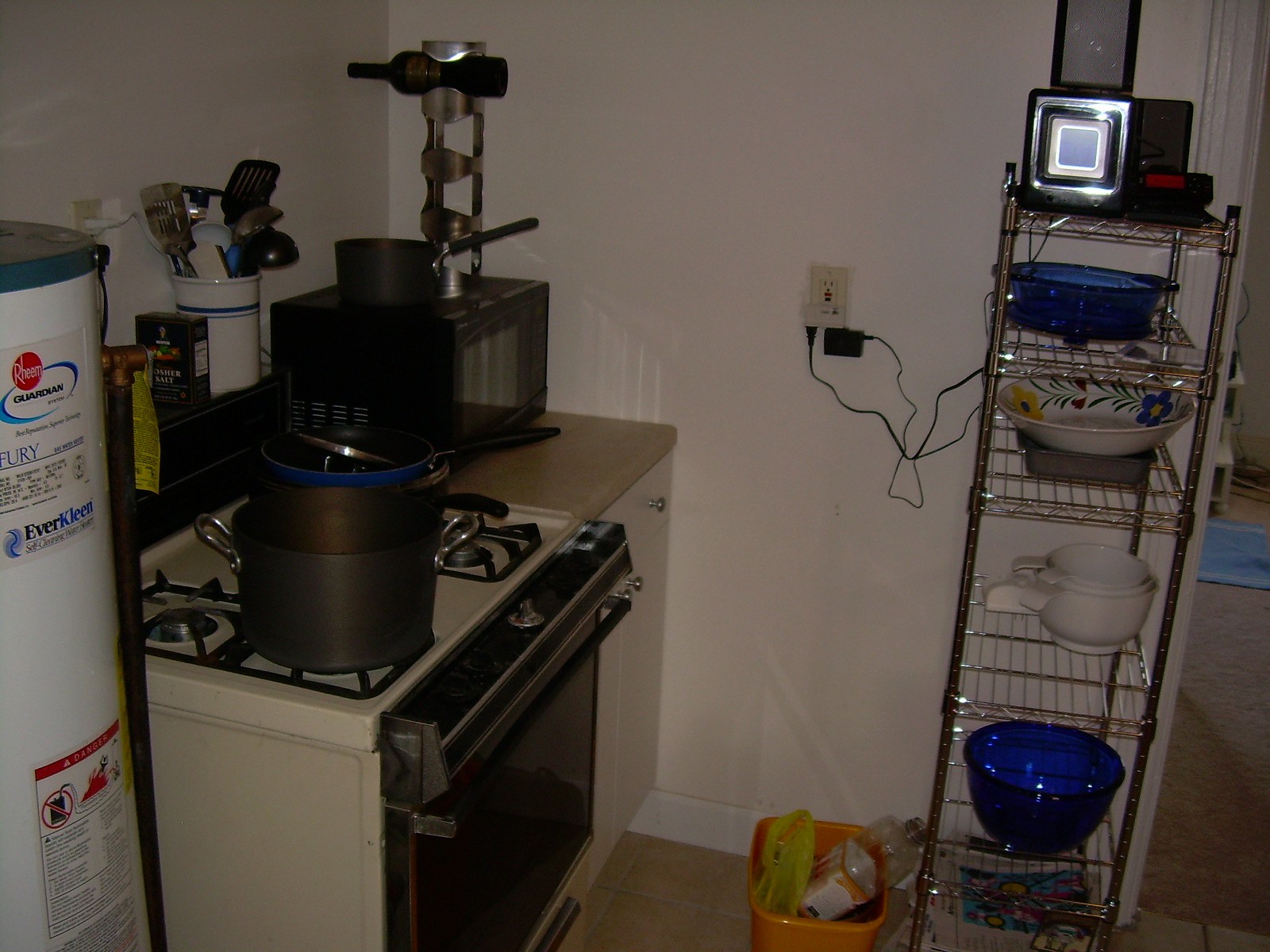The image depicts a detailed view of a cozy kitchen corner. Central to the scene is a cream-colored gas range, featuring both a stovetop and an oven, and topped with a stack of assorted pots and pans. Adjacent to the range on the right is a small countertop with a laminate, brown-colored surface. This countertop supports a microwave, another pot, and a wine holder containing a single bottle of wine. Behind the stove, a pot filled with kitchen utensils and a box of salt are positioned conveniently for cooking. To the left of the stove, there is a "Guardian" water heater manufactured by Ream Heating and Plumbing. In the foreground, a small square wire rack serves as a shelving unit, holding various bowls and kitchen materials. Atop this rack sits an electronic device, possibly a radio or stereo player, adding a touch of modern convenience to the kitchen space.